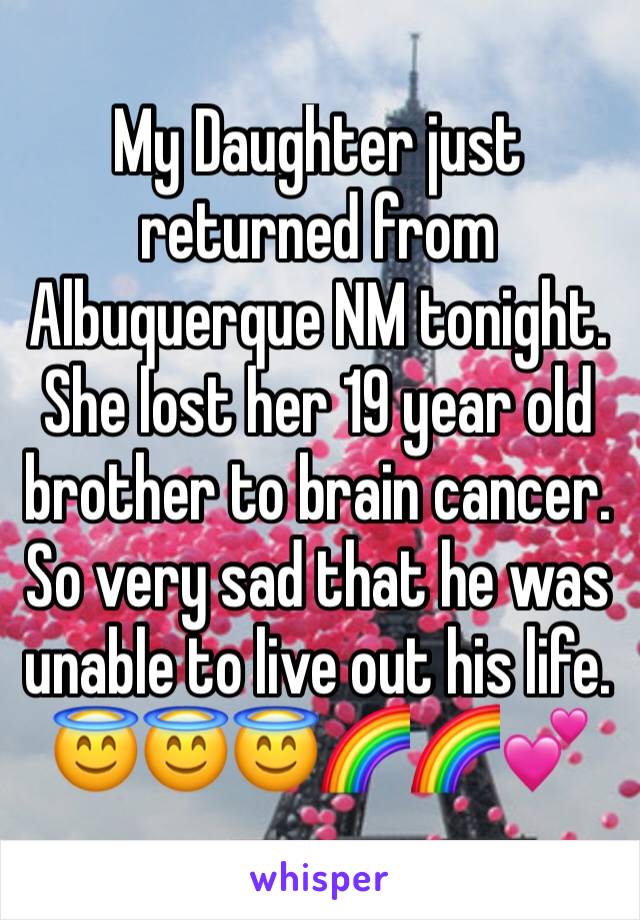The image appears to be a meme or social media post featuring a visually striking background and poignant text. The background prominently showcases the Eiffel Tower set against a cloudy sky, with an abundance of pink balloons framing the scene. Colors in the image include blue, white, black, gray, pink, yellow, and a spectrum of the rainbow such as red, orange, yellow, and indigo. 

The central text, written in white with a black outline in a fairly generic font, reads: "My daughter just returned from Albuquerque, New Mexico tonight. She lost her 19-year-old brother to brain cancer, so very sad that he was unable to live out his life." Beneath this heartfelt message, there are a series of emojis: three smiley faces with halos, two rainbows, and a double pink love heart. At the bottom of the image, the word "Whisper" is displayed in purple, indicating it was created using the Whisper app. The Eiffel Tower and balloons are slightly off-center to the right, while the text remains mostly centered, enhancing its legibility and emotional impact.